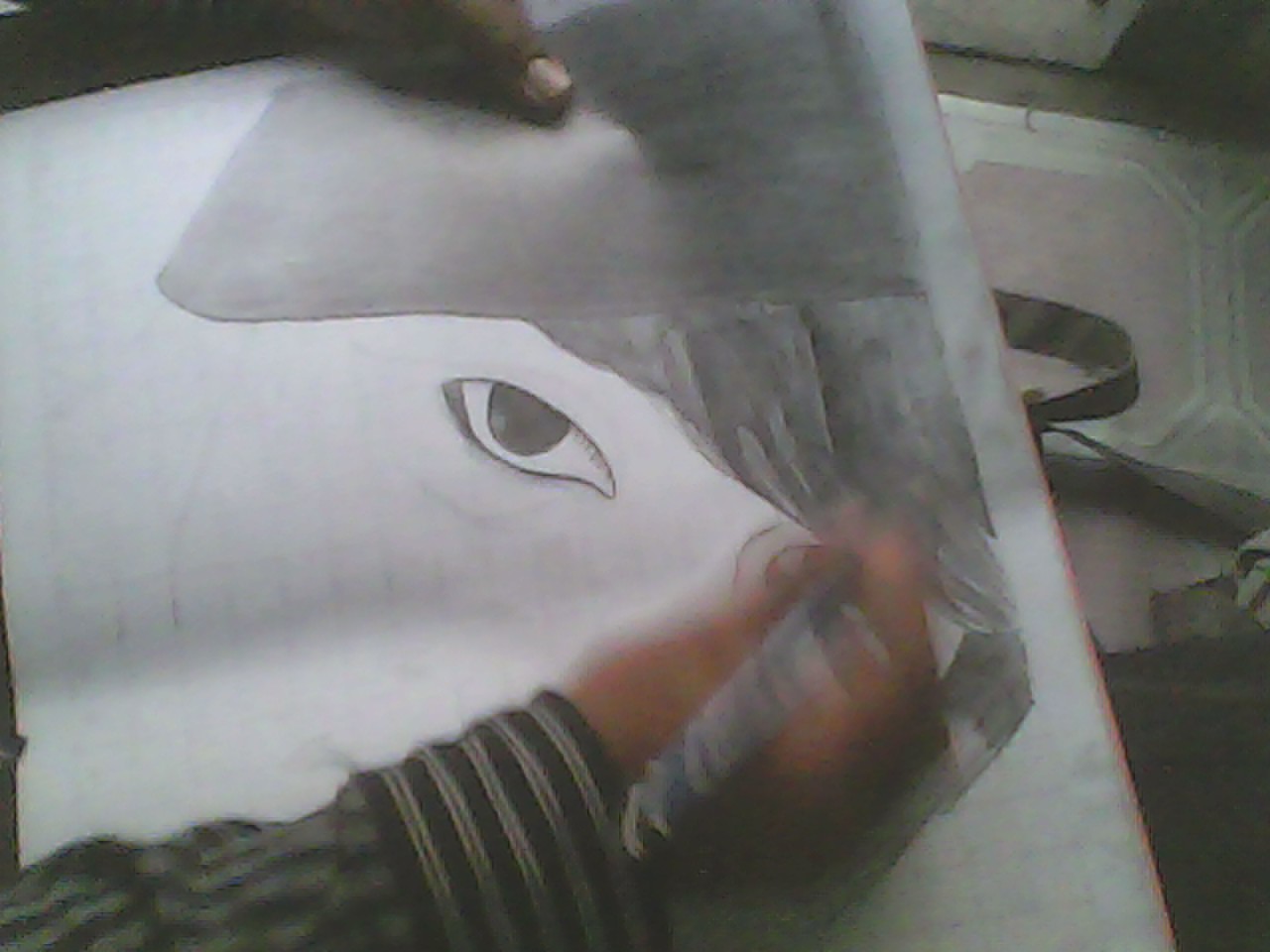A blurry image captures an artist in the midst of drawing on a large sketchpad resting on their lap. The artwork portrays the early stages of a human figure, identifiable by a detailed, black-colored eyeball and the beginning of black hair at the top. The artist's left hand and a portion of their right hand are visible, both holding a pencil, though the image clarity is low. They are donning a black and white striped long-sleeve dress shirt. In the background, a binder can be seen, but the overall setting remains indistinguishable. The absence of other people and text in the image shifts the focus solely onto the artist's meticulous work in progress.